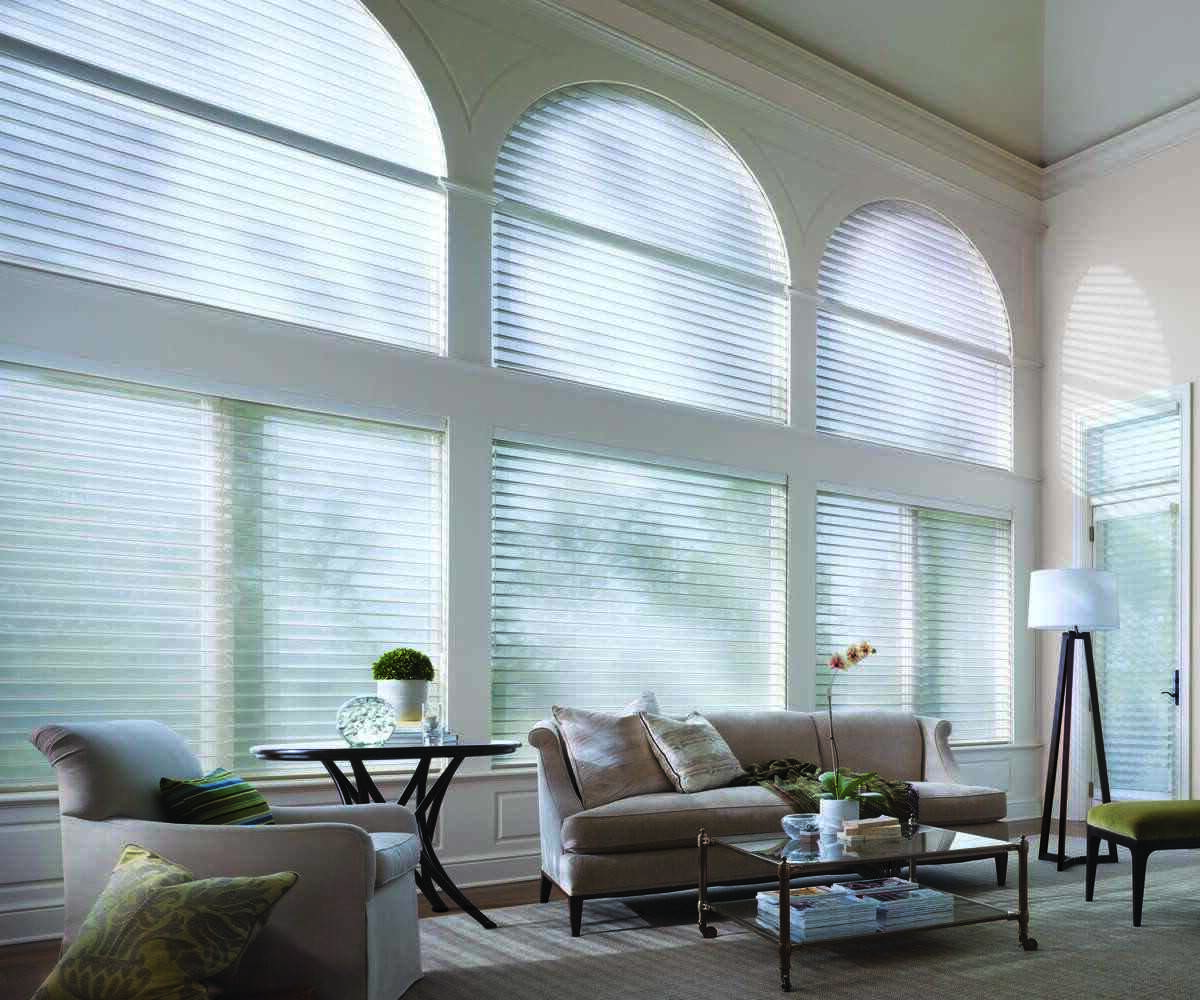The photograph captures an expansive, brightly-lit living room with impressively high ceilings. The focal point of the room is a wall adorned with large, multi-level windows that allow abundant daylight to stream in. The lower section of the wall features vertical rectangular windows, divided by slim wall partitions, while the upper section boasts rounded, dome-shaped windows, further enhancing the room’s airy atmosphere.

On the left side of the image, a white armchair with a green throw pillow sits invitingly, facing towards the right. Next to it, slightly further back, is a round wooden end table. Adjacent to the table is a light-colored sofa, adorned with a couple of throw pillows. In front of the sofa stands a glass coffee table, which holds a small plant and a few other objects, contributing to the room’s stylish yet cozy aesthetic.

To the right of the sofa, near the corner of the room, there is a standing lamp with a white shade. Completing the seating arrangement, the edge of an ottoman is just visible on the right side of the image. The walls of the room are white, and the bright, clear natural light from the windows illuminates every detail, creating a welcoming and serene living space.